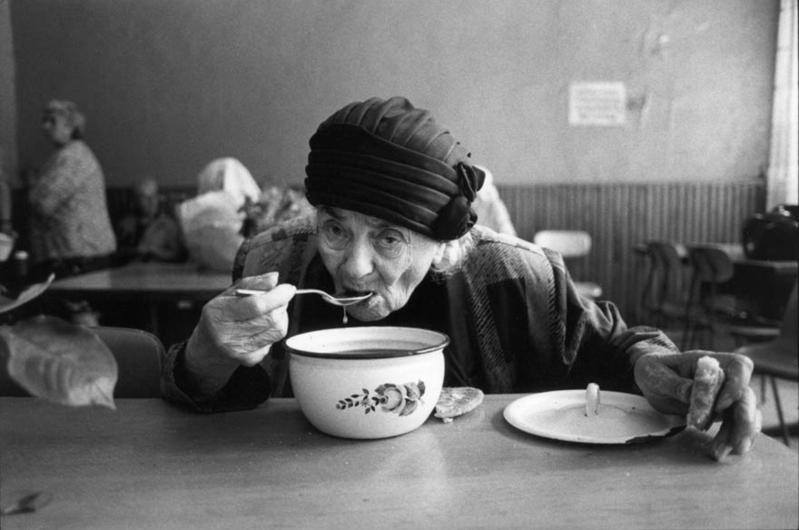In this black and white photograph, we see an older woman, reminiscent of a grandmother, deeply immersed in eating from a large, white, floral-patterned bowl of soup. The woman is wearing a black hat that wraps around her head in a style reminiscent of the 1920s. She is bent over the bowl with her mouth open, sipping from a spoon she holds in her right hand, a droplet of soup visibly falling back into the bowl. In her left hand, she clutches a small piece of bread. The bowl, which has a lid placed next to it, is set on a table. The woman's expression appears distant, as if she is going through the motions of eating without much thought. Her gaze seems unfocused, adding a sense of introspection or detachment. Behind her, another woman stands, and to her left, a small plant is visible on the table, contributing to the domestic atmosphere of the scene. The photograph, though monochromatic, vividly captures the moment in a detailed and evocative manner.